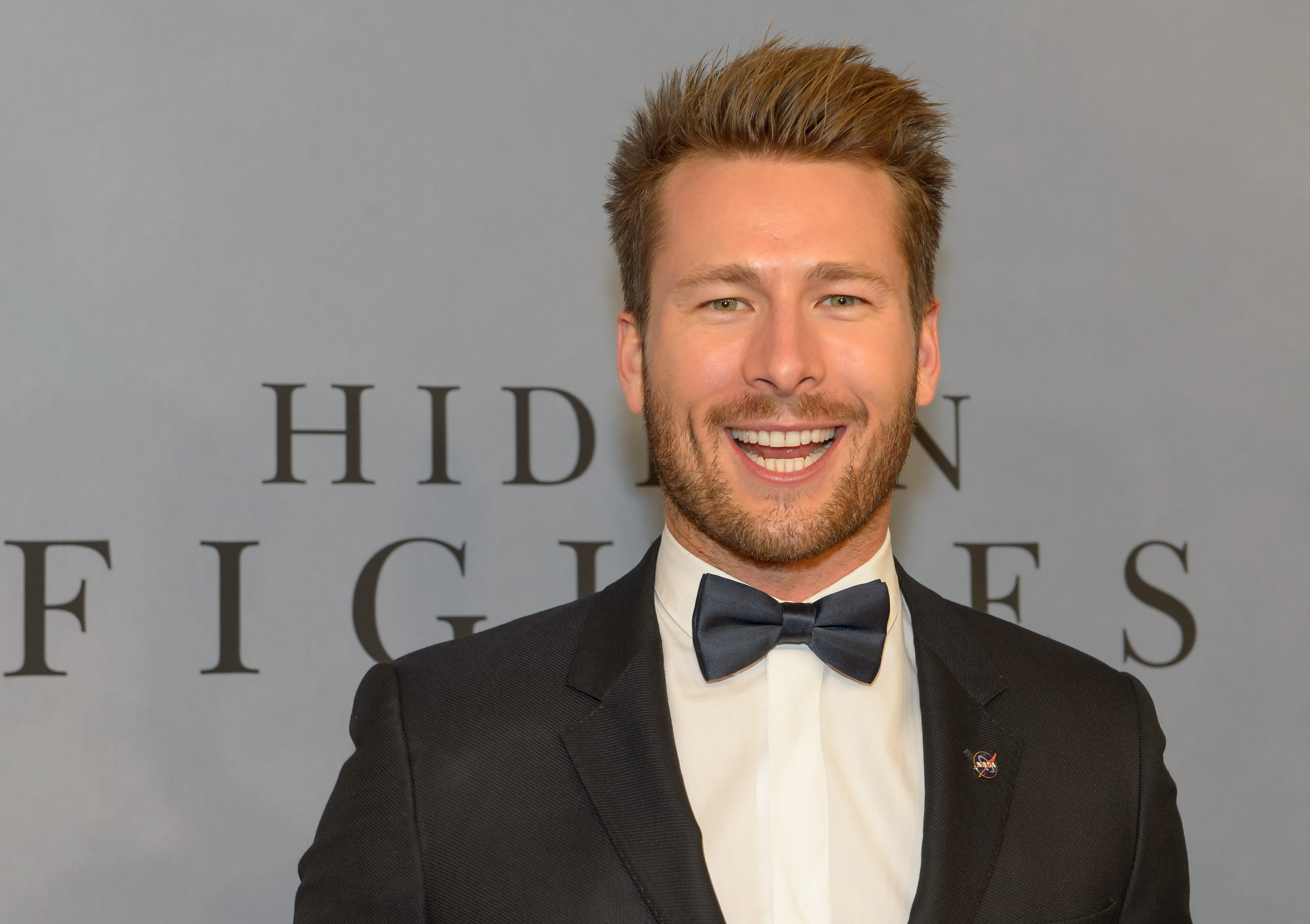The image depicts a young man with a big smile, dressed in a black tuxedo with a white undershirt and a black bowtie. He has spiky, light brown hair, a blonde mustache, and a beard. A pin with the NASA logo adorns one of his lapels. He stands positioned slightly to the right of center.

In the background, there is a light grey banner with prominent black text that reads "HIDDEN FIGURES." The text is partially obscured, with some letters more visible than others. The setting appears to be an awards ceremony or a special event. Notable colors in the image include light brown, dark bluish-gray, white, black, red, and tan.